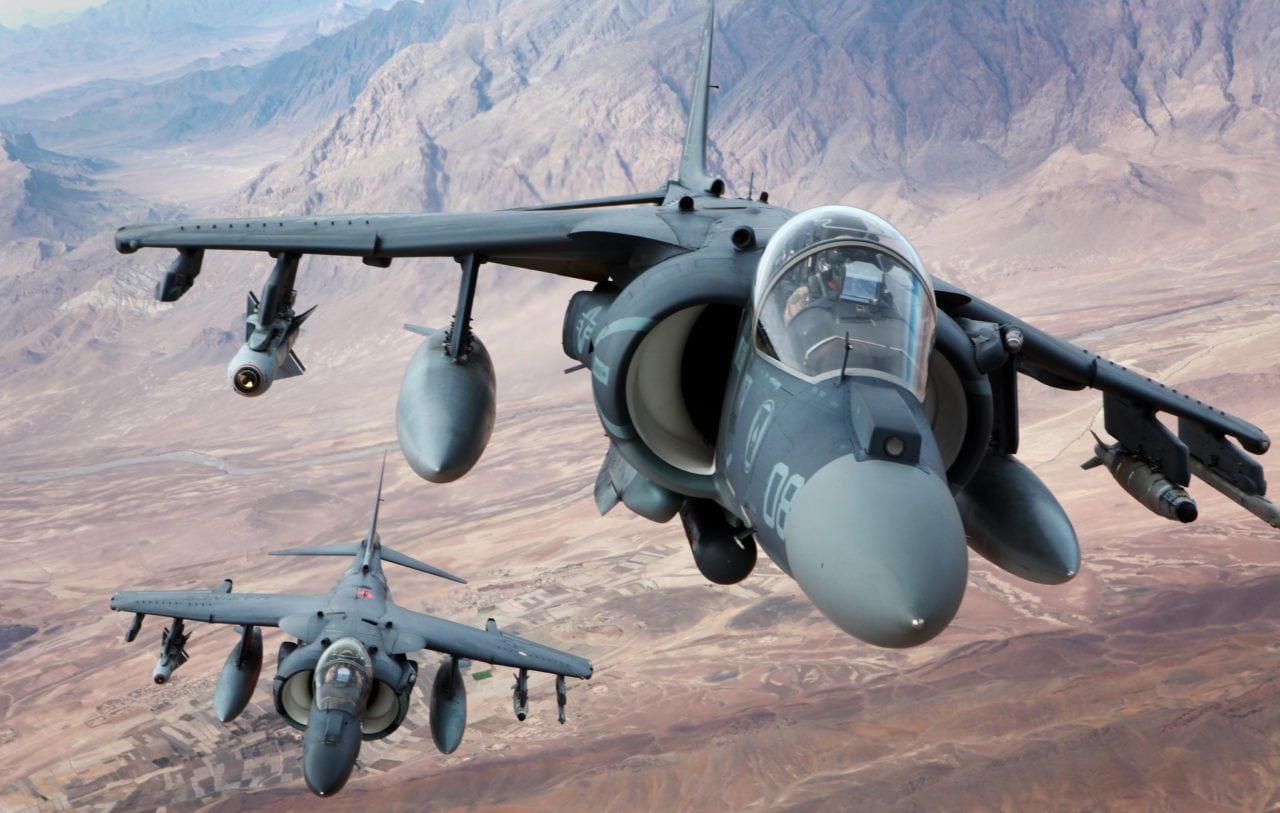The photograph captures an aerial scene of two similar gray and dark gray military fighter jets flying over a rugged, desert-like mountainous terrain. The foreground jet, larger and closer, displays the number "08" on its side and is equipped with missiles and jet engines. Its transparent cockpit reveals a glimpse of the pilot inside. This jet is skewed to the right, appearing almost as if it's heading towards the viewer. The second jet, positioned lower and further to the left, mirrors the first in design and equipment, including its aerodynamic shape and missile loadout, but appears smaller due to its distance. Both aircraft are set against a backdrop of brown, rocky mountains, which enhance the dramatic and dynamic nature of the scene.